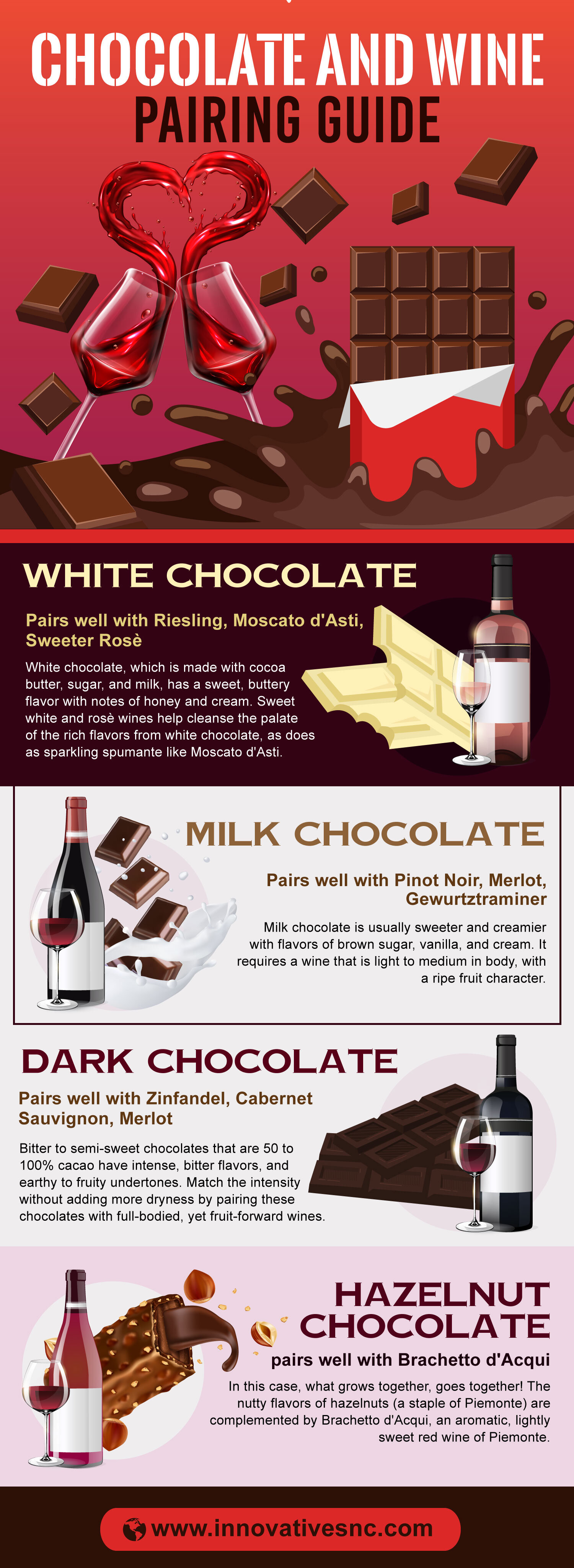This color infographic titled "Chocolate and Wine Pairing Guide" features a detailed, visually appealing advertisement that is organized into three main sections. At the top, in white text, it says "Chocolate and Wine Pairing Guide". Illustrations of two wine glasses clinking together create a splash that forms a heart shape, set against a reddish background with chocolate illustrations. 

The first section highlights "White Chocolate" and "Milk Chocolate". An image of white chocolate bars, some with bite marks, is paired with a wine bottle and glass filled with pink liquid, indicating Riesling, Moscato D'Asti, Sweet or Rosé wines. Next to it, the milk chocolate pairing section features squares of milk chocolate alongside a wine bottle and glass filled with red liquid, suggesting Pinot Noir, Merlot, or Gewurztraminer wines.

In the second section, "Dark Chocolate" and "Hazelnut Chocolate" are detailed. The dark chocolate pairing shows two bars of dark chocolate with a wine bottle and glass filled with dark red liquid, recommending Zinfandel, Cabernet Sauvignon, or Merlot wines. The hazelnut chocolate section depicts a piece of bite-marked hazelnut chocolate with a wine bottle and glass filled with red liquid, suggesting Bracero d'Aqui wine. 

Throughout the infographic, there are dynamic splash marks and flying squares of chocolate, enhancing the sense of movement. At the bottom, emerging from a pool of chocolate, is a partially unwrapped chocolate bar with splash marks around it. The visual elements conclude with a ribbon of chocolate and two hazelnuts. 

The advertisement finishes with a black rectangle at the bottom displaying the URL "www.innovativesnc.com" in red highlighted text.